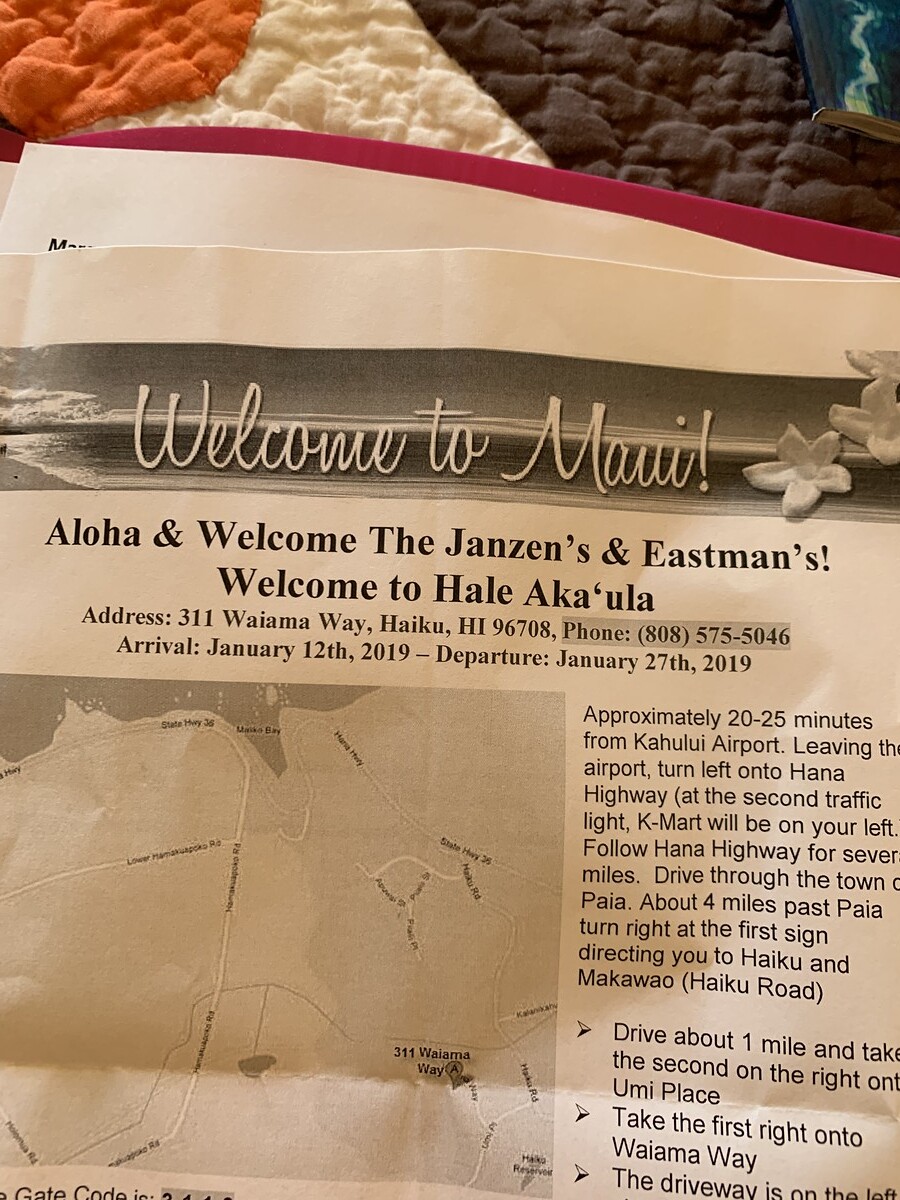The image depicts a flyer, printed in black and white, placed on a colorful quilt with brown, white, and orange patterns. The flyer welcomes the Jansons and Eastmans to Maui, stating "Aloha and Welcome the Jansons and Eastmans" and "Welcome to Hale Akaula." It includes detailed information such as the address "U.S. 311 Wai'amawe Haiku, Hawaii 96708" and the phone number "808-575-5046." The flyer specifies the arrival date as January 12, 2019, and the departure date as January 27, 2019. Turn-by-turn driving directions from Kahului Airport are meticulously listed, guiding visitors through landmarks such as Kmart and the town of Paia, finally leading to Waimai Way. To the left of the written content is a printed map, possibly sourced from Google Maps or a webpage, showing the route visually. The paper appears to be lying on a quilt, sometimes described as brown, white, and orange, and other times referred to as laying on a red folder or quilt. Lastly, small flower drawings decorate the flyer to the right of the opening greeting.